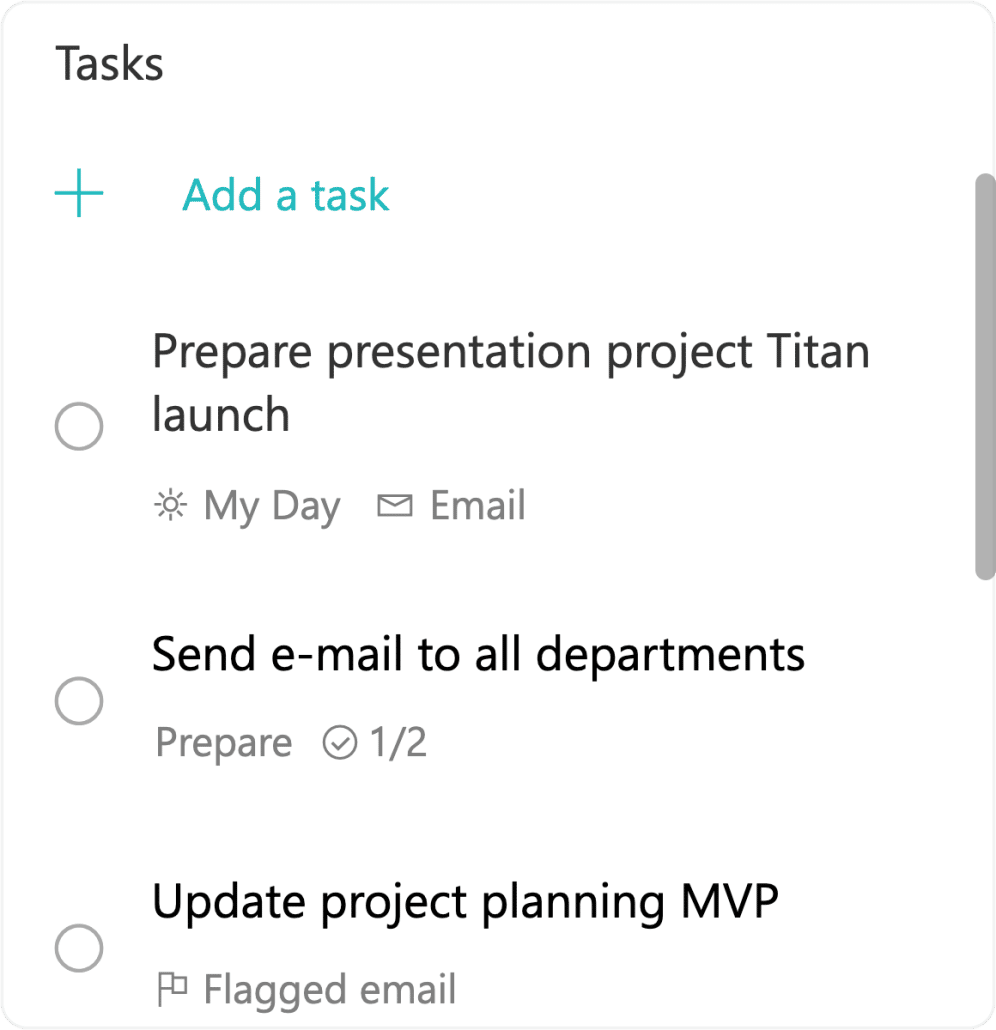Here is a detailed and refined caption for the described image:

---

The image is a vertically-oriented rectangle with rounded corners, bordered by a faint gray line. A dark gray scrollbar extends from about a third of the way down on the left-hand side. At the very top, the header reads "Tasks" with a turquoise plus sign labeled "Add a task" beneath it. 

Below the header, the first task entry has a circular radial button with a gray outline and white center next to the text "Prepare Presentation for Project Titan Launch." There is a sun icon labeled "My Day," followed by an envelope icon and the word "Email."

The second task entry, mirroring the previous style, is "Send Email to All Departments." It also features a circular radial button, and adjacent to it, a smaller circle containing a progress indicator marked "1/2."

The final task at the bottom reads "Update Project Planning MVP," again accompanied by a similar radial button. To its right is a small flag icon with the text "Flagged Email." 

The entire background of the image is white, providing a clean and minimalistic design.